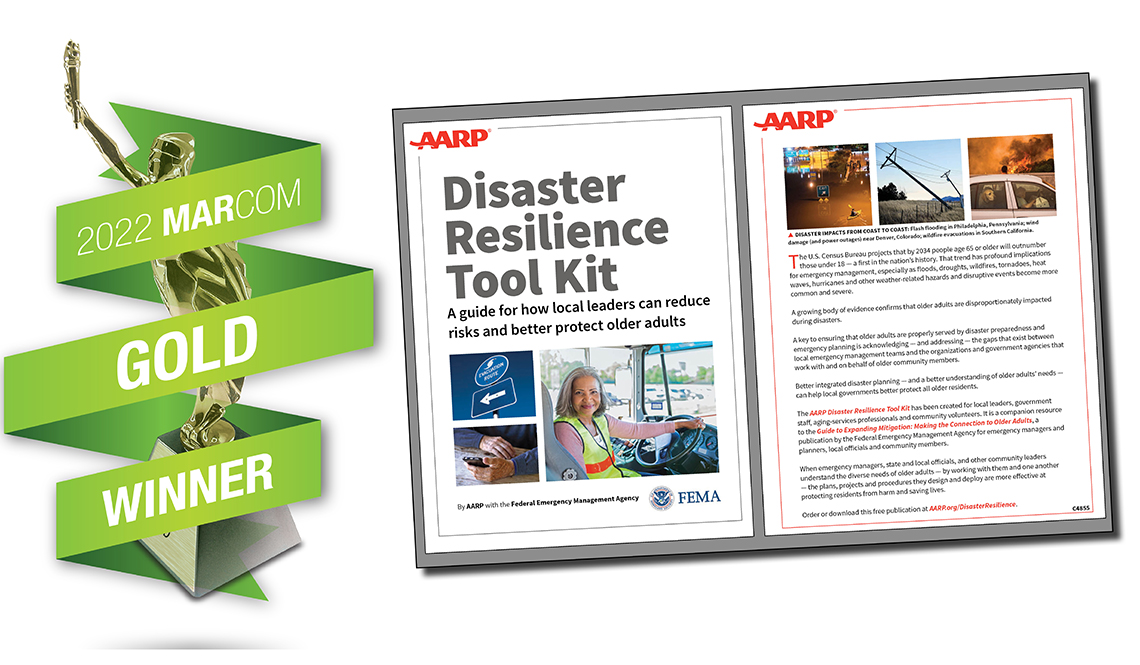The image is designed to promote workplace safety among businesses. At the center, two A4-sized sheets of paper are displayed side by side within a grey border, each featuring an "AARP" logo in red font at the top left corner.

The left sheet prominently showcases a large headline reading "Disaster Resilience Toolkit" in black font, occupying nearly half of the page. Beneath the headline, a subtext explains that this toolkit is "a guide for how local leaders can reduce risks and better protect older adults." Following this description, there are three images arranged vertically: a road sign, a person's hands using a smartphone, and a woman in a high-visibility vest sitting at the wheel of a large vehicle.

The right sheet begins similarly with the "AARP" logo in red at the top left corner. It features three images at the top – one depicting downed power lines, another showing people inside a car, and a third image that is indistinct due to its small size. The rest of the sheet is filled with detailed paragraphs of black text, interspersed with highlighted red text to emphasize key points.

Flanking these sheets is a gold statue adorned with a green ribbon, labeled "2022 Marcom Gold Winner." This trio of elements is set against a plain white background, enhancing focus and readability.

In summary, the visual arrangement on a white background aims to underscore AARP's commitment to enhancing safety and resilience for businesses, especially targeting the protection of older adults.